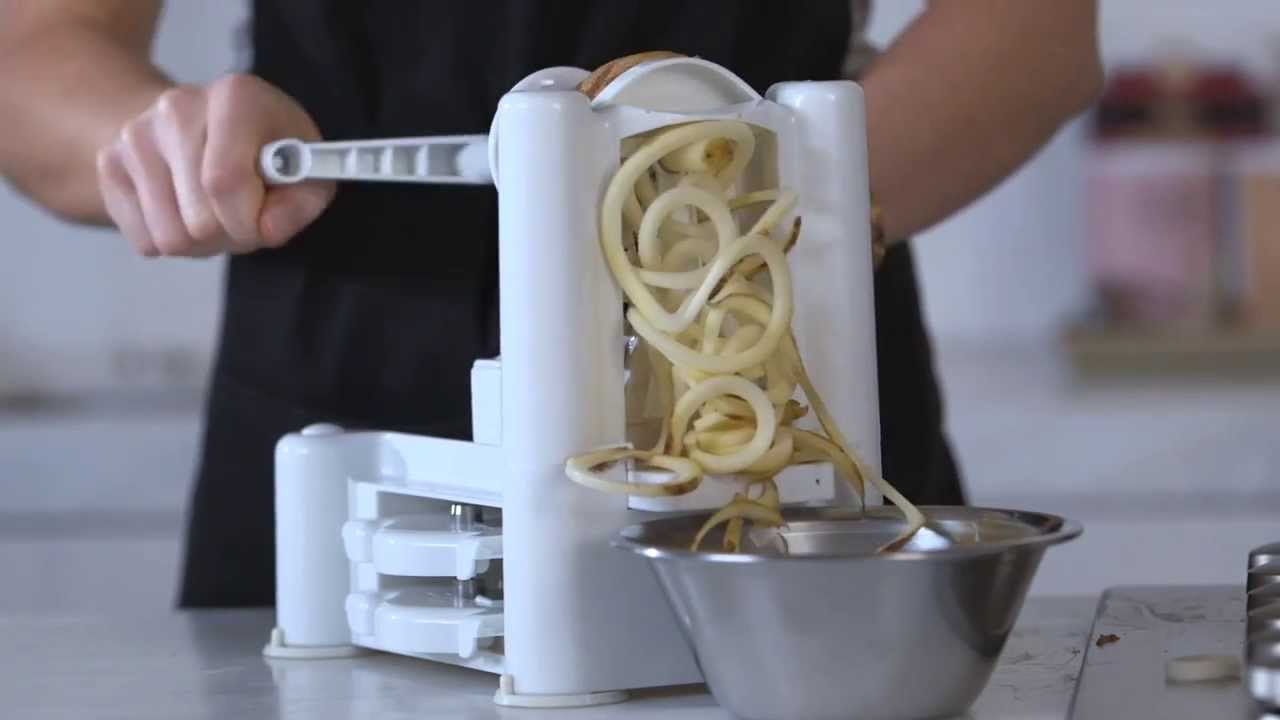The image depicts a close-up view of a person, seen from the waist up, operating a small kitchen appliance designed to create curly fries or spiralize vegetables. The individual is dressed in a black outfit, which could be a black dress or apron, and is actively turning a crank attached to the white plastic machine. The appliance is positioned on a table and features two small circular poles at the front, a handle at the top, and a platform at the bottom. As the person turns the handle, lengthy strands of yellow potato, stripped of their brown skin, emerge from the front end of the machine. These potato spirals descend toward a stainless steel bowl placed in front of the appliance, ready to catch the processed potato strings. The appliance, largely white with some visible metal screws, appears functional but somewhat cheaply made. The overall setup is straightforward and situated against a white background.